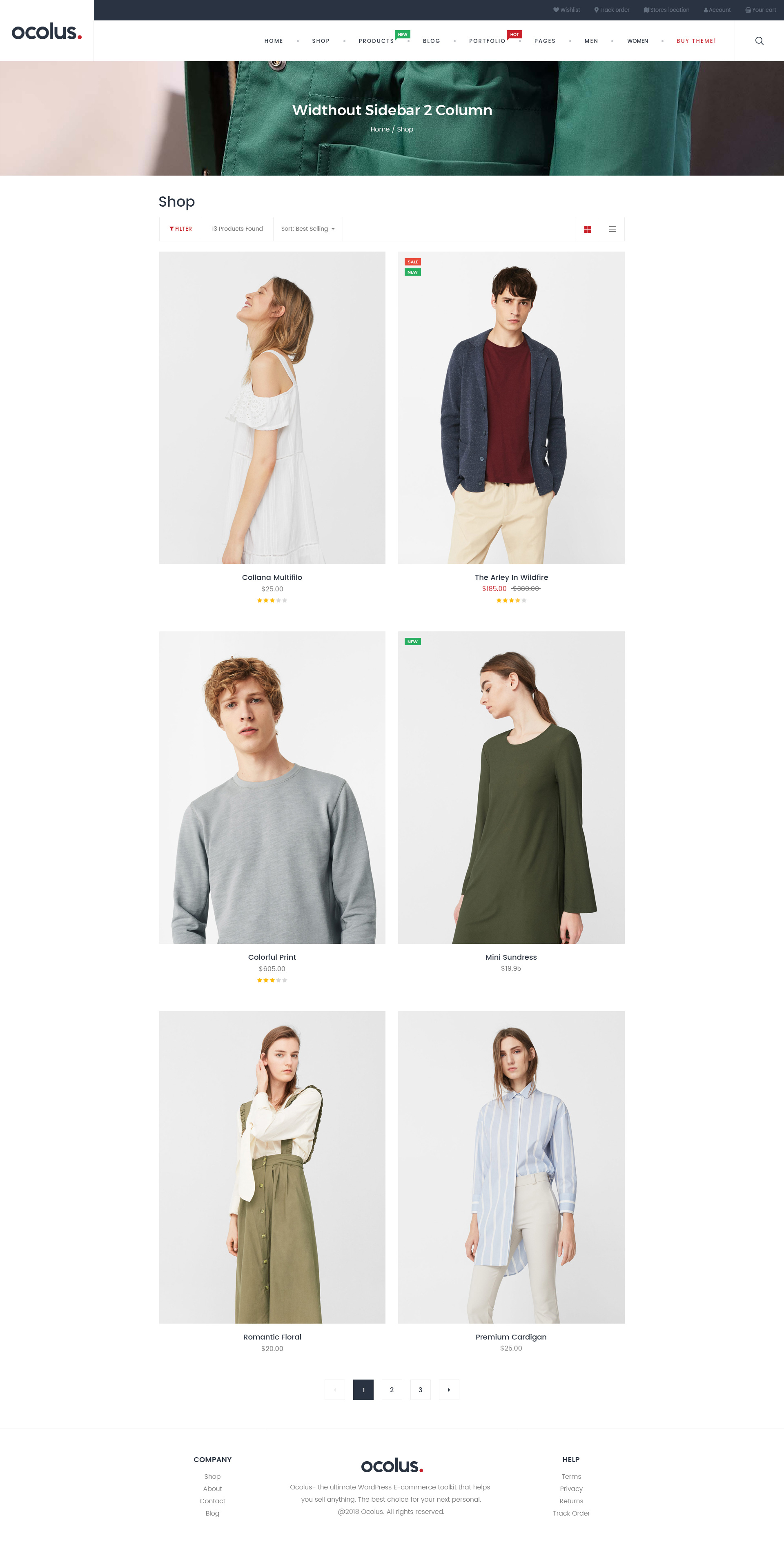**Caption:**

Oculus Fashion E-commerce Website Layout

The image captures a detailed view of an e-commerce website for a fashion store named "Oculus" (not to be confused with the virtual reality company). The top navigation bar includes links such as Home, Shop, Products, Blog, Portfolio, Pages, Men, Women, and utility links like Wishlist, Track Order, Store Location, Account, and Cart.

Prominent action buttons on the website are labeled "New," "Hot," "Buy," and "Theme." The main content area features a banner layout without a sidebar and is organized in a two-column format with a breadcrumb trail labeled "Home / Shop."

In the shop section, there are filter and sort options visible, indicating that 13 products have been found. Users can sort the products by "Best Selling" and toggle between different product layout views, including a grid view.

The displayed products include:
1. **Colanda Multi El Nino**: Image of a woman in a white dress, priced at $25 with a 3-star rating.
2. **The Arley and Windfire**: Image of a man in a blue cardigan, on sale for $18 (originally $30), with a 4-star rating.
3. **Colorful Print**: Image of a man in a gray sweatshirt priced at $65, with a 3-star rating.
4. **Mini Sundress**: Image of a woman in a green dress priced at $19.95, with a 5-star rating, marked as new.
5. **Romantic Floral**: Image of a woman in a green and white outfit (pants or dress) priced at $20, with a 4-star rating.
6. **Premium Cardigan**: Image of a woman in a blue and white striped shirt and white pants priced at $26, with a 5-star rating.

Pagination links for navigating to different pages (1, 2, and 3) are located at the bottom of the page. The footer contains links to Shop, About, Contact, and a description about Oculus stating it as the ultimate WordPress e-commerce toolkit for selling anything, touted as the best choice for your next personal project. Copyright information is provided, indicating "2018 Oculus All Rights Reserved."

Note: This is not associated with the well-known Oculus brand related to virtual reality.